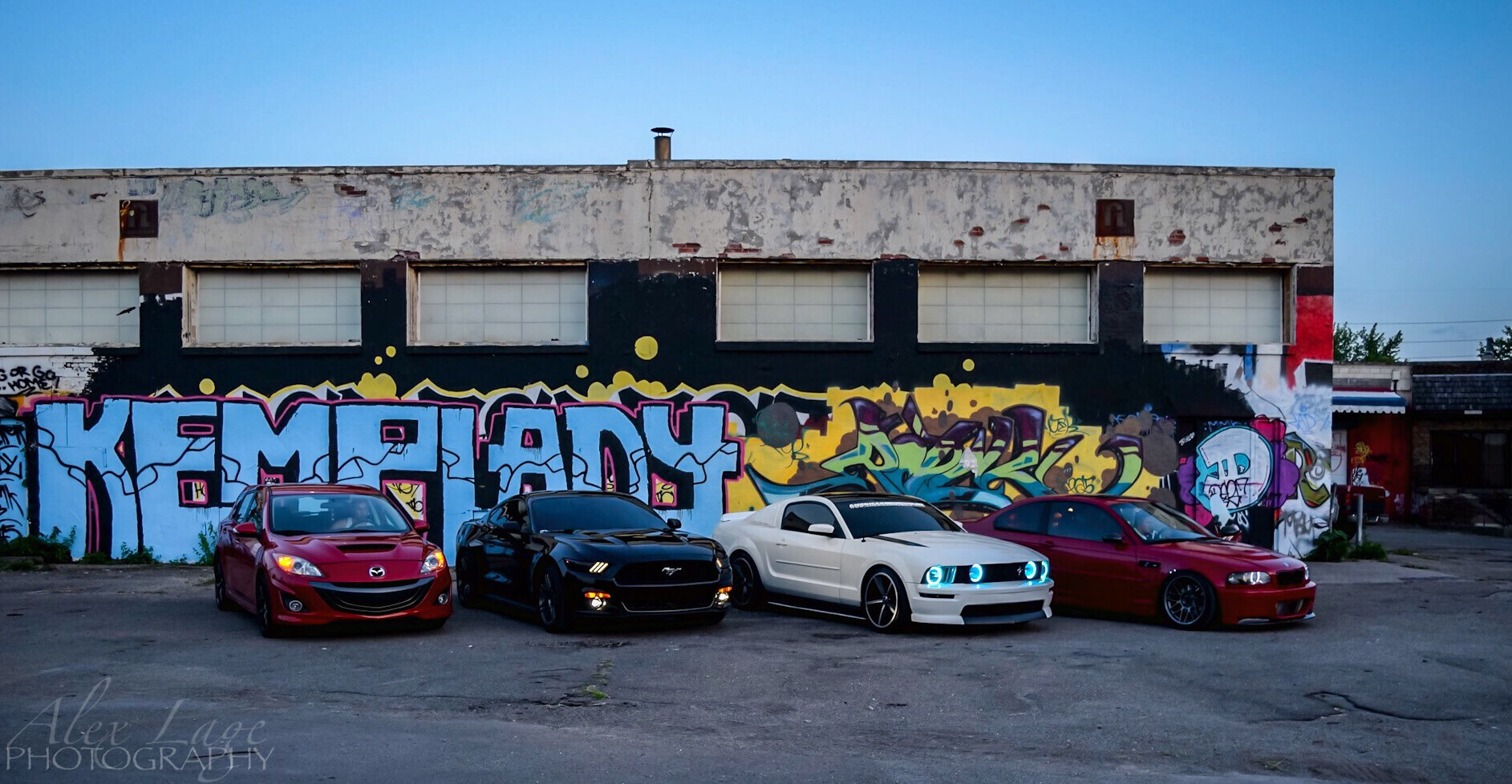In this detailed horizontal image, four sporty, muscle-type cars are parked side-by-side in front of a large, flat-topped building with several large rectangular windows near the top. The windows are covered with a light tan-colored material, preventing visibility inside. The upper part of the building's facade exhibits a weathered, marble-like gray and tan surface, while the lower two-thirds to three-quarters of the wall is painted black and adorned with vibrant graffiti. The graffitied text includes blue bubble letters spelling "KEMP LADY," interspersed with yellow, green, white, purple, and red bubble designs. A single vent is located at the upper center of the building. The sky is a clear blue, highlighting the outdoor setting.

The cars, lined up slightly at an angle to the right, display their headlights; they are colored red, black, white with a black hardtop, and red, from left to right. The car to the far left has a visible occupant, while the interiors of the other three cars are not clearly visible. The street they are parked on is cracked and poorly maintained, adding to the gritty, urban atmosphere. On the bottom left of the photograph, there is a watermark reading "Alex L-A-G-E Photography," marking the photographer's credit.